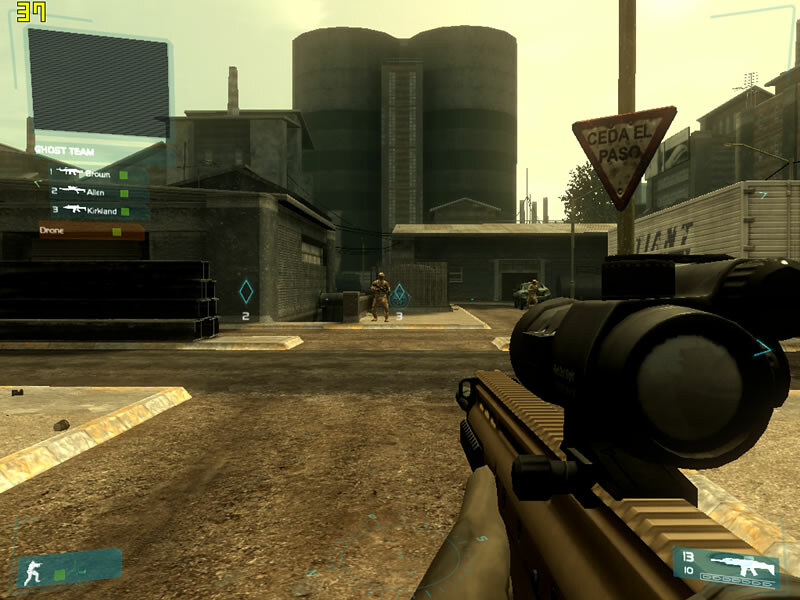The image is a detailed screenshot from a first-person shooter video game. The main focus is on a character in the game holding a large military-style assault rifle with a prominent scope, aimed at a distant man. There are tall gray buildings in the background, one of which has a sign that reads "Cita El Pasa," indicating a Spanish-speaking setting. The top of the screen displays the number 37 in bright yellow. The lower left corner features a small blue box with a character and a green health bar partially filled, while the lower right corner shows icons and a count of 13 shots and 10 rounds remaining. Additional interface elements include another blue box on the right possibly depicting an airplane, and a game board with unclear icons. The left side of the screen lists team members—Brown, Allen, and Kirkland—under "ghost team." The setting appears industrial with the presence of silos, a tractor-trailer, and an abandoned factory-like atmosphere.